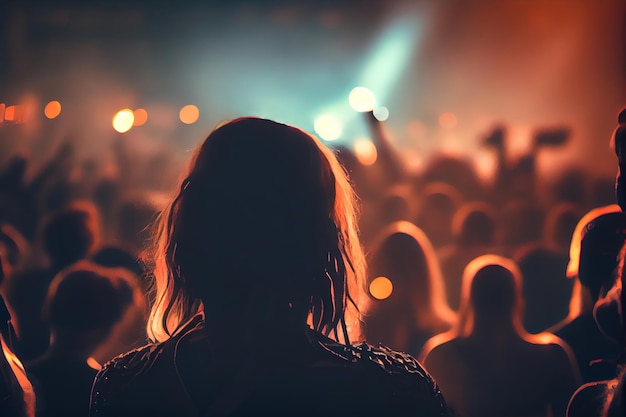In this shadowy concert scene, the photograph (possibly AI-enhanced) focuses on the back of a woman’s head, her shoulder-length hair softly illuminated by a subtle orange hue from the stage lighting. She stands amid a bustling crowd, all facing the stage where the lights dance in shades of orange and blue. The image is intentionally blurred at the peripheries, drawing attention to the intricate details of her hair while leaving the faces of the crowd and specifics of the stage in obscurity. Glimpses of hands raised in the air and lens flare effects add to the lively, almost surreal atmosphere of the live concert.